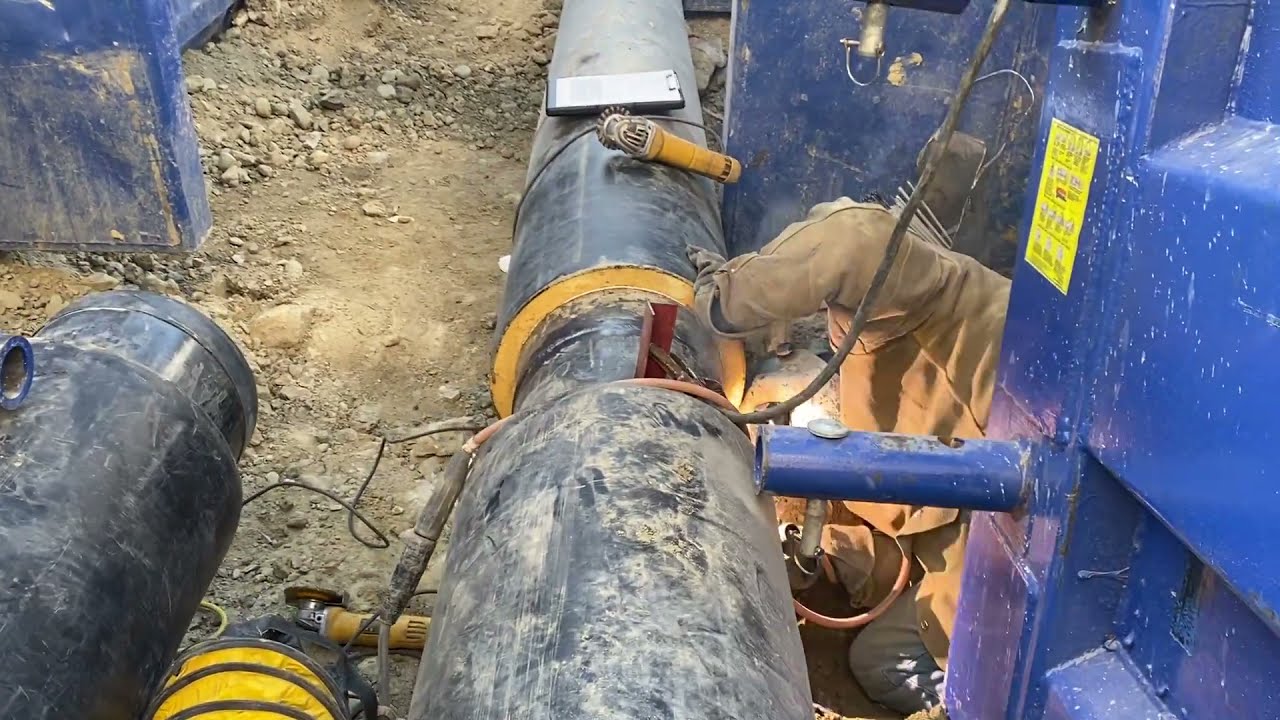This detailed image captures an active construction site focused on pipeline work. At the center of the scene runs a large pipe extending from the foreground towards the rear, situated amidst a landscape of exposed dirt and rocks in a tannish-beige hue. A person, potentially involved in welding, is partially visible, identifiable possibly by the elbow and knee, clad in a tan Carhartt jacket, blue jeans, and likely equipped with a welding mask that glows slightly, suggesting ongoing work.

To the bottom left, another black pipe with yellow-bordered ends and black ribs encircling it emerges, accompanied by additional tubular structures nearby. A blue framework or wall stands on the right, dotted with yellow labeling and dirt, and features scattered clevis pins.

Several handheld tools – black, yellow, and silver in color – are strategically positioned on and around the central pipe. One tool resembles a cutting instrument, another appears more like a grinder, and a third item, possibly a clipboard, lies behind the central tool. Black cables, some draping over the pipes, contribute to the bustling industrial environment, indicative of complex and detailed technical work being performed.